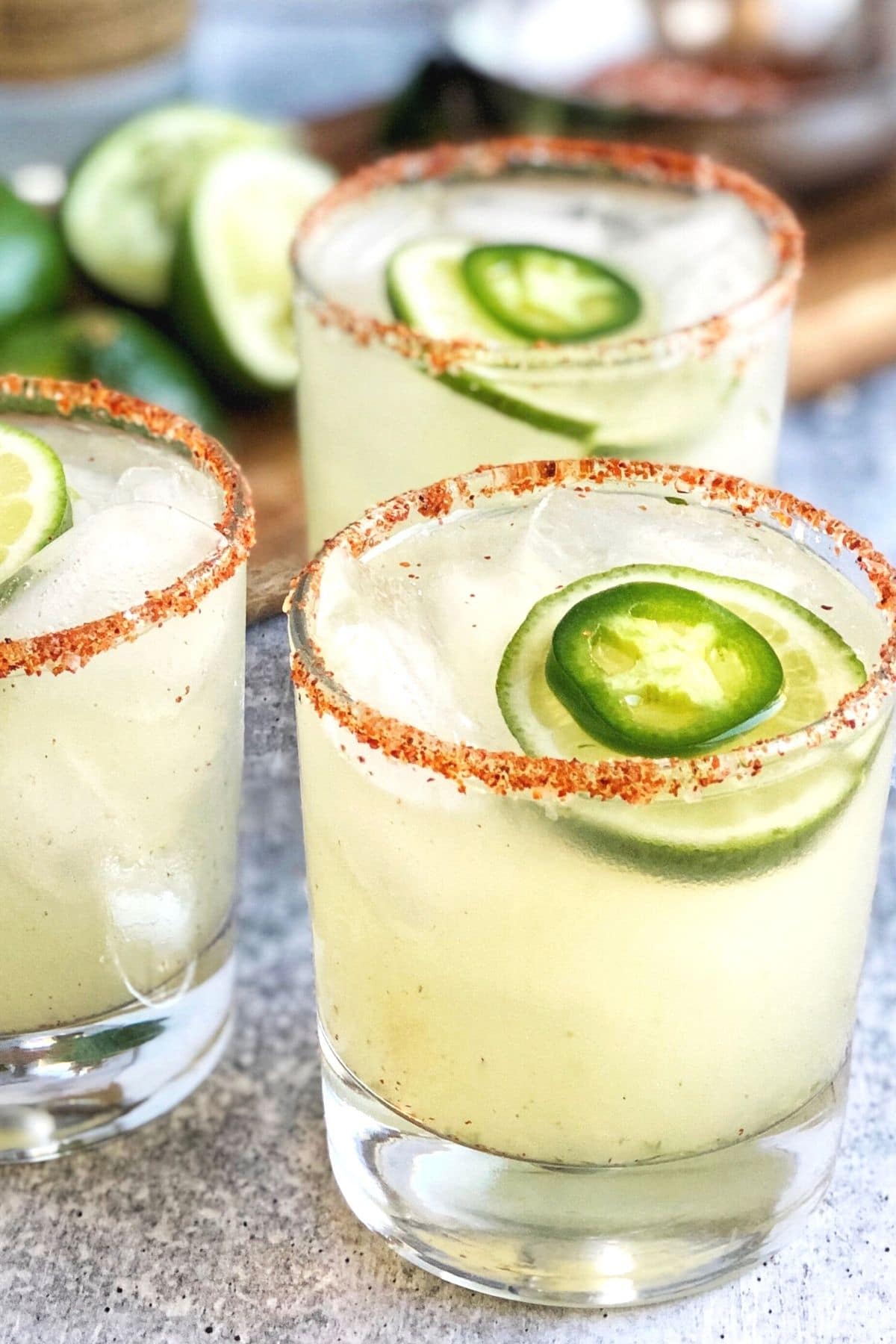This photograph captures three small glasses filled with what appears to be a spicy margarita, set against a granite table. The glasses, which hold about six ounces of liquid, are short and round with a thick base visible beneath the pale yellow, lime-colored drink. Each glass is garnished with a slice of lime and a small slice of jalapeno floating atop rock ice, and their rims are coated with a reddish chili spice blend, likely comprising tajin and salt. The background features a cutting board with sliced limes, slightly blurred to keep the focus on the drinks. The image is devoid of people and hands, emphasizing the vibrant, spicy cocktails as the main subject.